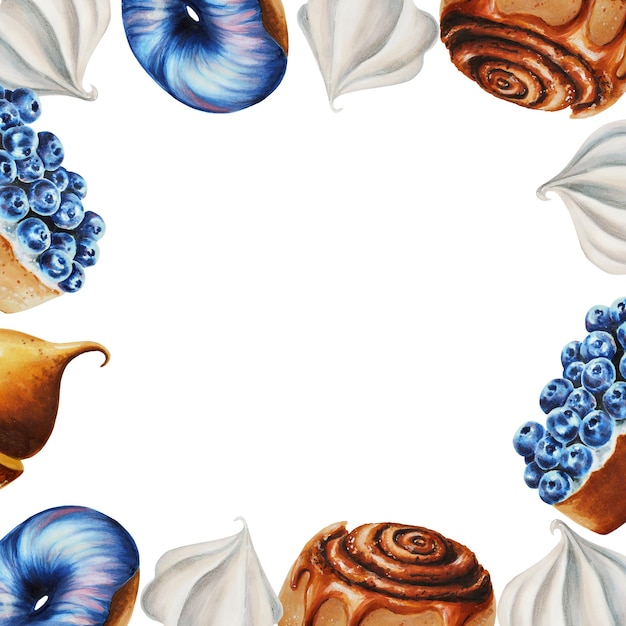This square-shaped, 5-inch by 5-inch image is set against a plain white background and prominently features an intricate arrangement of pastry drawings facing inward around the border. In the top right-hand corner, there's a detailed illustration of a brown cinnamon roll drizzled with chocolate icing. To its left hangs a creamy dollop of vanilla soft serve ice cream or meringue. Adjacent to this, a donut with vibrant blue and pink icing captures attention. The upper left-hand corner also showcases a puffy white dollop. Below it, a decadent cake topped with blueberries and scalloped white icing is depicted. Continuing downward, a rich brown dollop of ice cream adds depth. The lower left corner features another donut, this time with blue and purple icing, followed by another white dollop. The bottom right corner presents another cinnamon roll with chocolate icing facing upward. Above it, another white dollop is situated, followed by the blueberry-topped cake with white icing, and culminating at the very top with yet another white dollop. This food art piece with no accompanying text uses a harmonious palette of browns, blues, purples, and whites to vividly showcase desserts like cinnamon rolls, donuts, ice cream, and cakes, all arranged intricately around the piece's periphery.